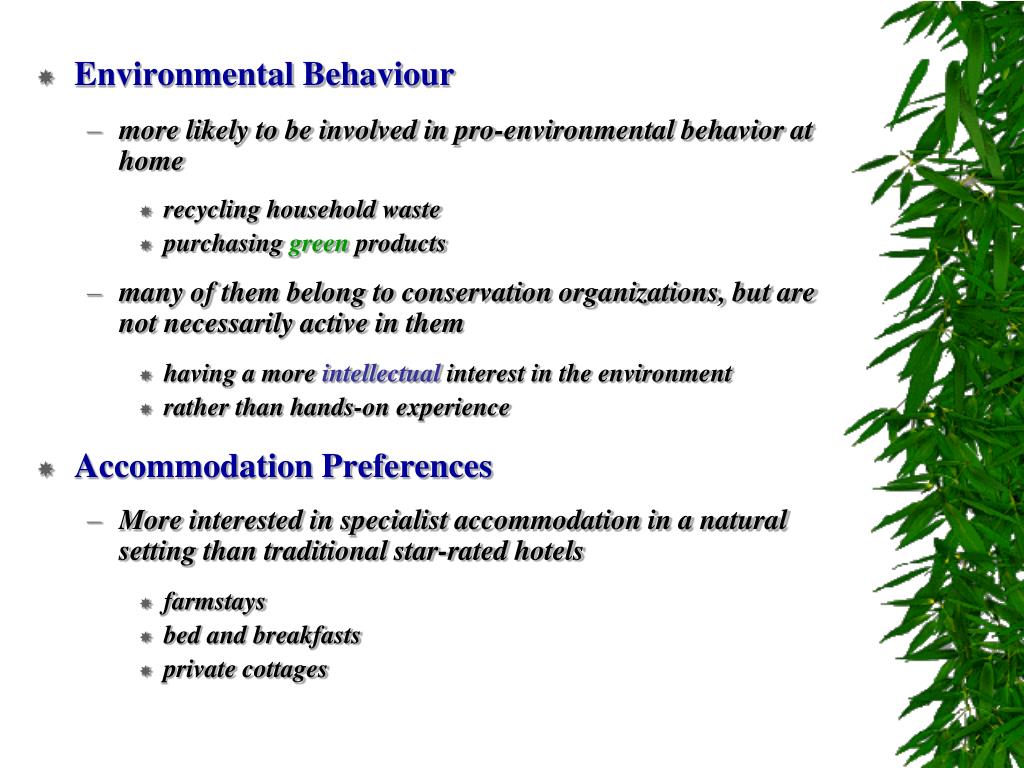This image features a predominantly text-based composition on a white background, with a strip of greenery extending vertically along the right-hand side. The greenery consists of narrow, dark green leaves that appear to be alive and attached to a plant, possibly resembling bamboo or a similar plant.

The text is organized into two main bullet points, each marked by an asterisk-like symbol in dark blue or purple, with capitalized headings. The first bullet point reads "Environmental Behavior," and the second one, positioned further down, reads "Accommodation Preferences."

Under "Environmental Behavior," several sub-points detail pro-environmental activities:
- The primary text states individuals are "more likely to be involved in pro-environmental behavior at home."
- Two smaller bullet points list specific behaviors: "Recycling household waste" and "Purchasing green products," with "green" written in green font.
- Another segment, marked by a hyphen, notes that "many of them belong to conservation organizations but are not necessarily active in them."
- Further sub-points elaborate on the environmental interest: "Having a more intellectual interest in the environment" (with "intellectual" in lighter purple) and "Rather than hands-on experience."

Under "Accommodation Preferences," the text reads:
- "More interested in specialist accommodation in a natural setting than traditional star-rated hotels."
- This is followed by three smaller bullet points listing preferred types of accommodation: "Farm stays," "Bed and Breakfast," and "Private cottages."

The structure and content suggest an informational pamphlet or digital document focused on environmental behavior and accommodation preferences, aimed at readers with a pro-environmental inclination.